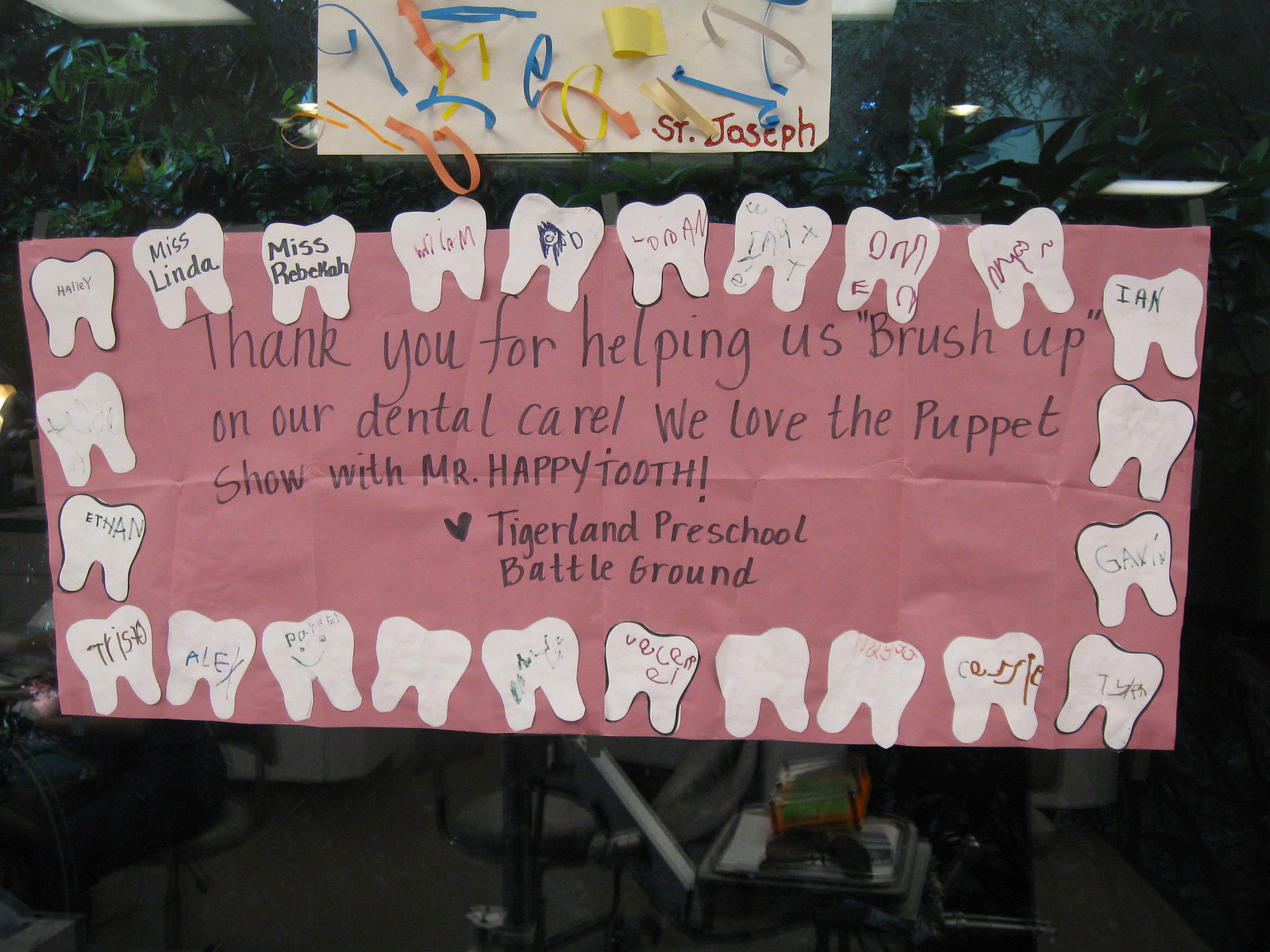This is a detailed photograph of a handmade, horizontally long rectangular banner-style poster, prominently purple in color. The poster features an array of white, rounded, paper cutouts resembling molars, each with a name written inside, such as Ian, Alex, Ethan, and Haley. The focal message, written on the purple background, reads: "Thank you for helping us brush up on our dental care. We love the puppet show with Mr. Happy Tooth." The banner is signed with love from Tigerland Preschool Battleground, and it includes the names of teachers Miss Linda and Miss Rebecca. The poster appears to be displayed in a classroom-like setting with plants and chairs visible in the background, suggesting a space filled with youthful activity and care.